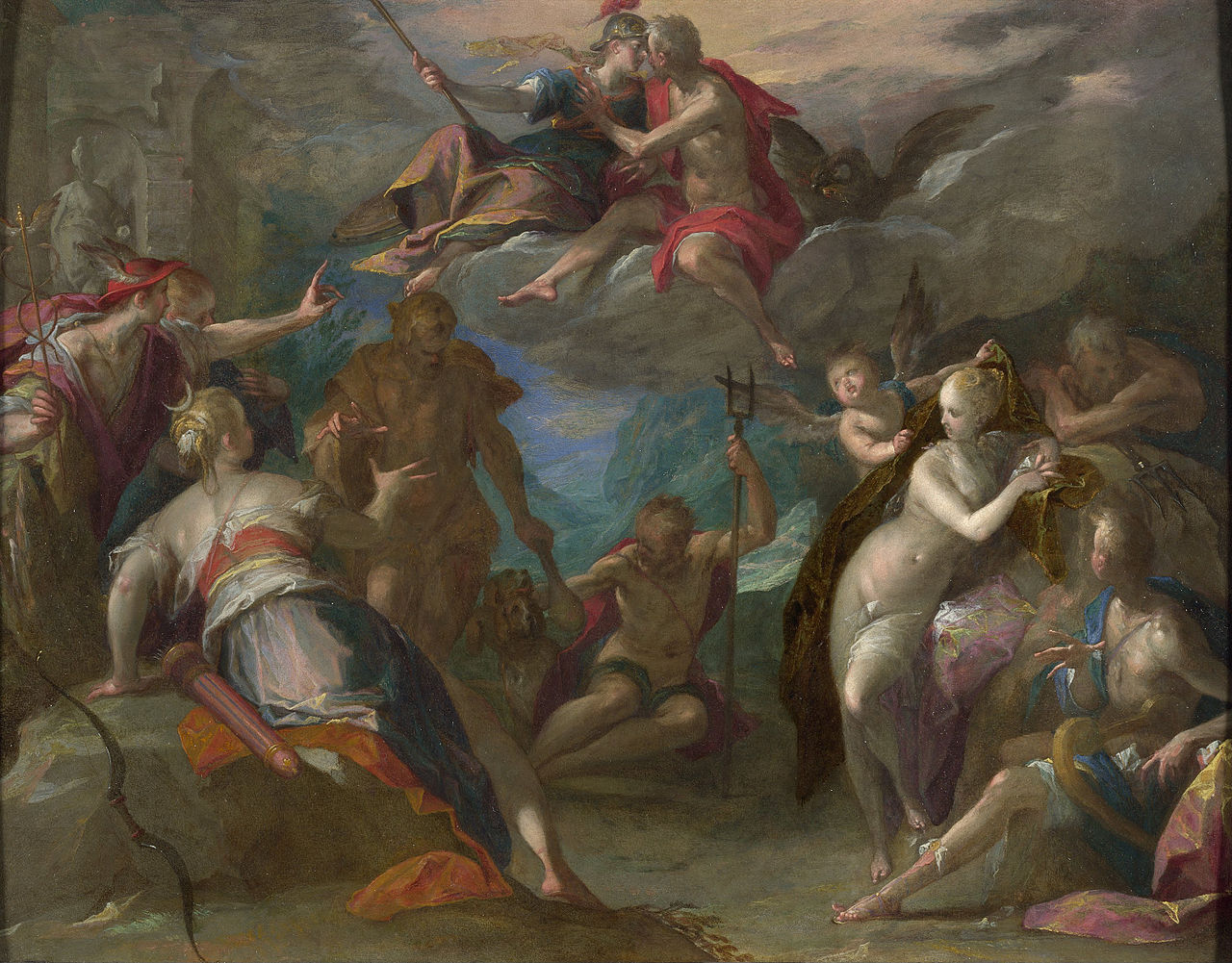This is a detailed Renaissance-era religious painting that captures a scene filled with turmoil and a quest for salvation. Dominating the heavens, two figures—a man and a woman, appearing to be on the verge of kissing—sit amidst the clouds. Alongside them, an angel and a bird further emphasize the celestial theme. Below, a group of people, both men and women in various states of undress, reach out towards the sky. The scene is accentuated by a small cherub with wings, adding to the painting’s religious overtones. A prominent figure sits on the ground in the middle, holding a pole and draped with a cloth for modesty, flanked by two dogs. The color palette is predominantly beige and white, with touches of blue, contributing to the overall atmosphere of turmoil and urgency.